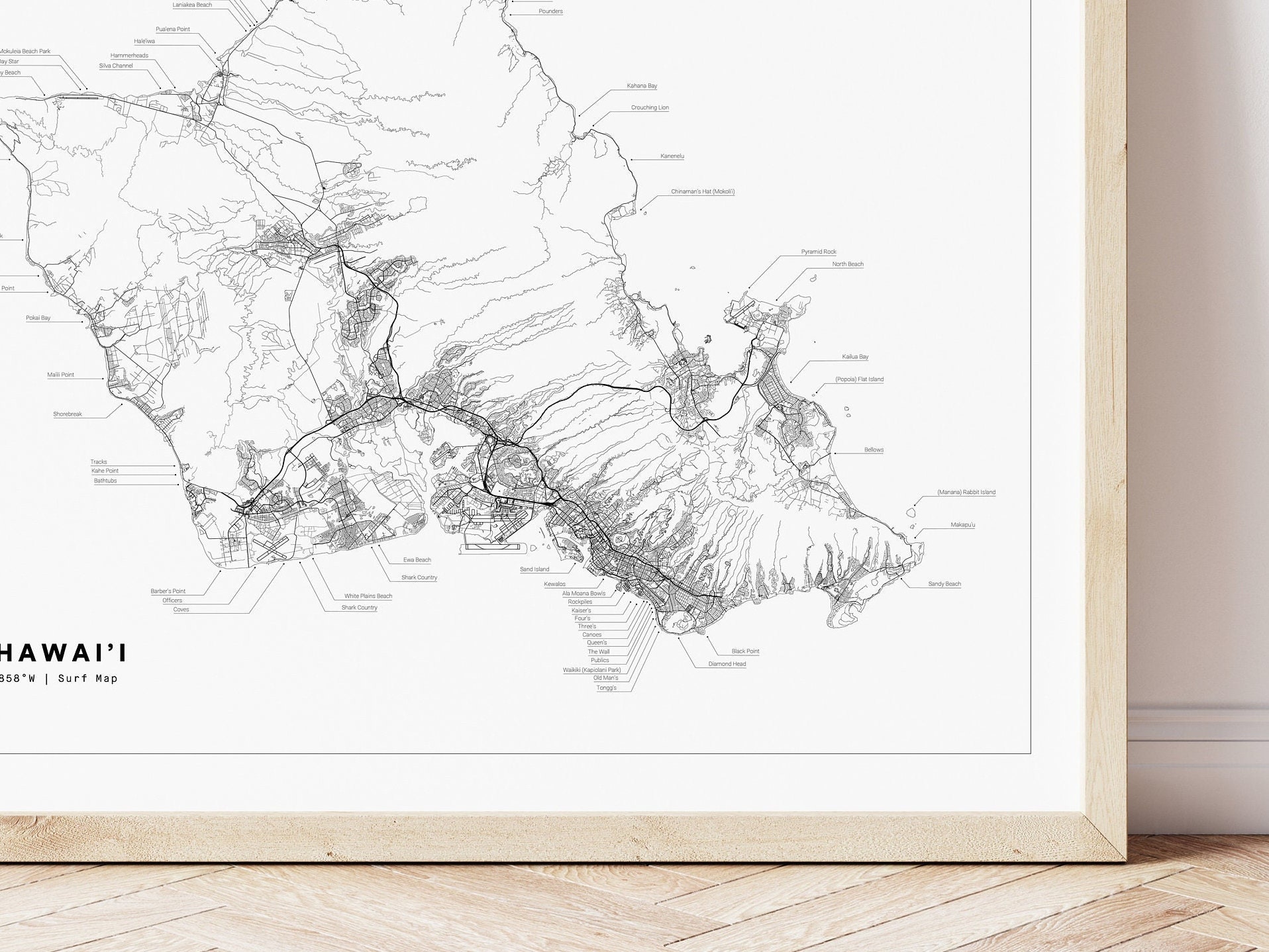The photograph features a closely cropped image of a frameless piece of art, propped up against a white wall and resting on a beige wood-like floor. The wall and frame both share a light wood color, contributing to the bright, white aesthetic of the scene. The centerpiece is a black and white line art map of the main island of Hawaii, depicted with intricate, fine print that is challenging to read from a distance. The map is labeled "Hawaii Surf Map" at the bottom, with the text surrounded by detailed annotations around the coastlines, likely indicating various beaches and surf spots such as Sandy Beach, Black Point, and Diamond Head. The map itself is bordered by a white matting, which enhances its clean and minimalistic design.